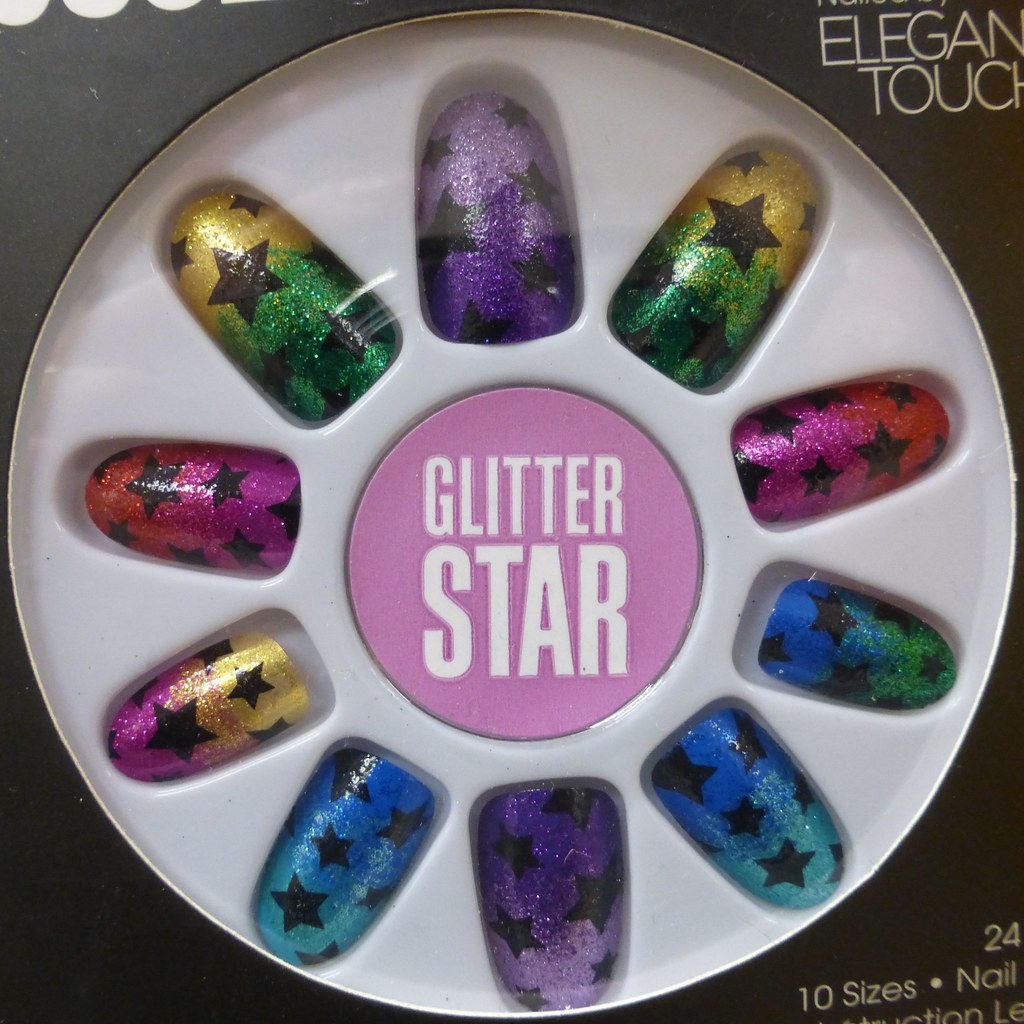The image depicts a package of colorful, glittery press-on nails arranged in a white circular tray with a pink center that reads "GLITTER STAR" in white, capital letters—STAR is notably larger than GLITTER. The tray features 10 different nail designs, each adorned with black star patterns and vibrant colors, including purple, green, yellow, red, and blue. At the top of the circle, there's a purple nail with dark stars, flanked by two green nails with yellow tips. Below, red sparkly nails with stars are followed by three blue nails featuring a green sparkle and stars, and a half red, half gold nail with stars. Another purple nail with dark stars completes the set. The surrounding package, on a brownish background, is partially cut off, displaying "ELEGANT TOUCH" at the top right, and "24 ten-sized nails" at the bottom right, though the numbers and some letters are obscured.